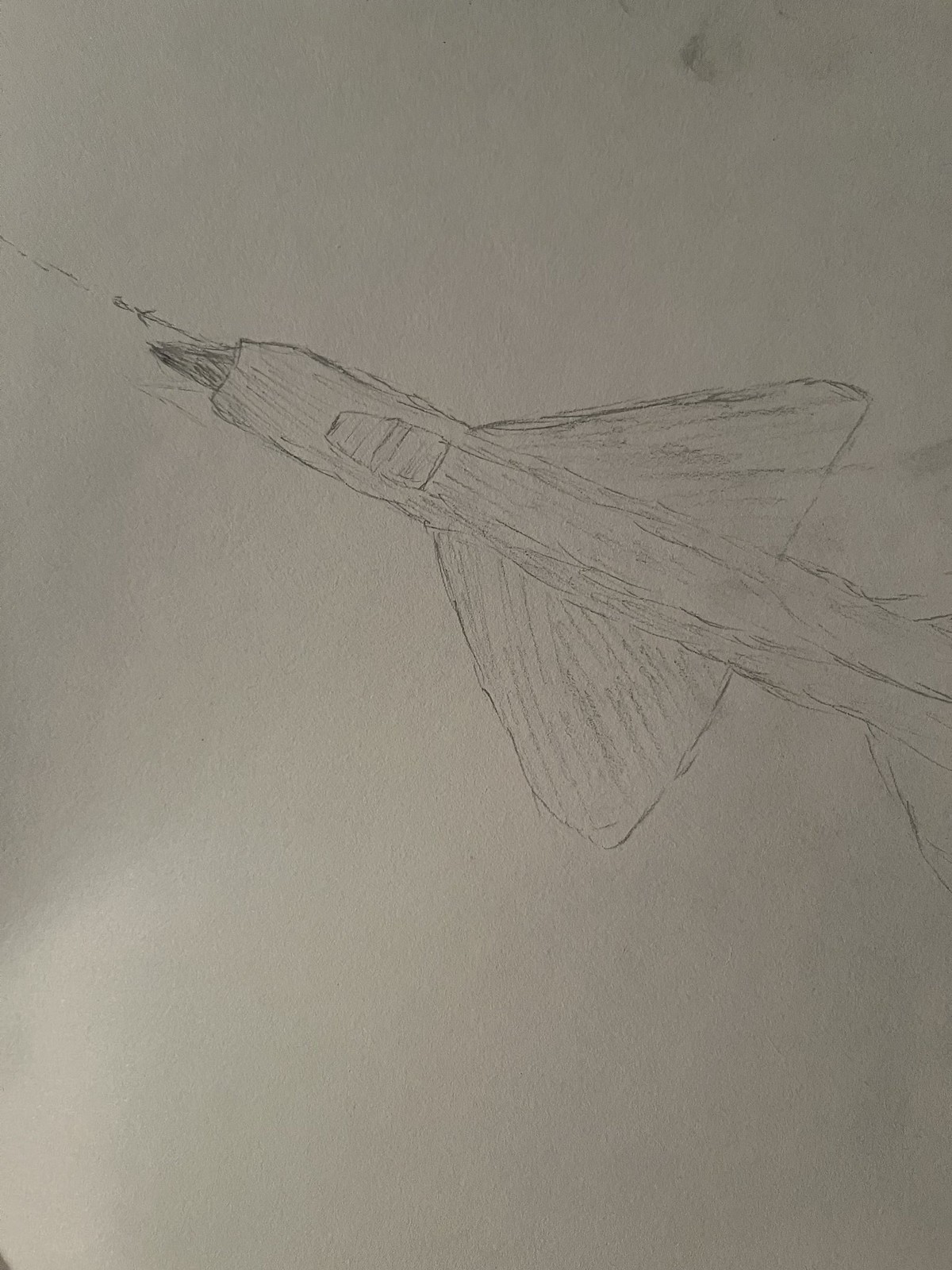This photograph captures a detailed pencil sketch on white paper, although the dim lighting gives the image a darker tone. The central figure in the sketch appears to be a rocket, characterized by triangular wings of equal size affixed to its sides and a pointed, darkened front. A notable jet stream emerges from the rear, typically indicative of propulsion. The sketch suggests a landing gear section and depicts a missile or bullet being launched from the rocket's nose, suggesting dynamic action. The perspective offered seems to be from the underside of this airborne vessel, showcasing intricate details of its design and function.